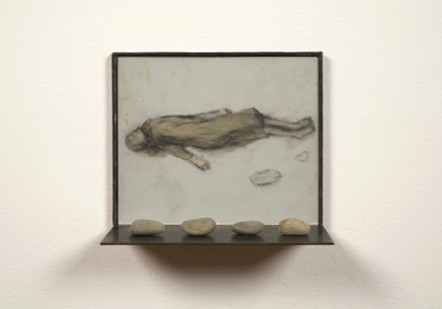The image is an art installation mounted on a plain off-white wall. At the bottom of this installation is a thin black ledge holding four smooth stones of equal size. The centerpiece of the installation is a square artwork with a black frame, featuring an illustration of a person lying flat on their back. This figure, sketched in green with a black outline, wears a long-sleeved shirt and a knee-length yellowish dress. They appear barefoot, with their head tucked back and arms resting by their sides. The background of the drawing is gray, and within the image are two irregular shapes that appear to be a big and a small rock. The wall beneath the installation casts a slight shadow, adding depth to the presentation.